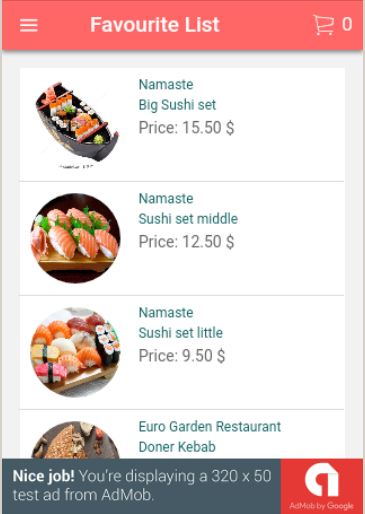Here is a detailed, cleaned-up caption based on the description provided:

---

This image appears to be a digital menu screen for a sushi restaurant. At the top, there's a red band. On the left side of this band, there are three horizontal white lines stacked above each other, indicating a menu icon. In the center, the text "Favorite List" is displayed, and on the right side, there's a shopping cart icon with the number "0" next to it, signifying that the cart is empty.

Below this banner, the menu showcases four items, each presented in white rectangles. The last item is partially cut off at the bottom of the image. 

1. The top item features an image of a sushi boat with the text "Namaste Big Sushi Set" priced at $15.50.
2. The next item shows a circular dish of sushi, labeled "Namaste Sushi Set Middle" priced at $12.50.
3. Below that, another circular dish with sushi is labeled "Namaste Sushi Set Little" priced at $9.50.
4. The partially cut-off item at the bottom indicates another restaurant, "Euro Garden Restaurant Donor Kebab."

At the very bottom of the screen, a gray strip is present with a congratulatory message: "Nice job! You displayed a 320 by 50 test ad from AdMob." To the right of this message, there is a red background area with the text "AdMob by Google" and a white icon, though this part is somewhat difficult to discern clearly due to its color contrast against the gray background.

The fonts used on the menu items are mostly in shades of green-blue or gray.

---

This caption provides a comprehensive and detailed description of the menu image based on the original input.